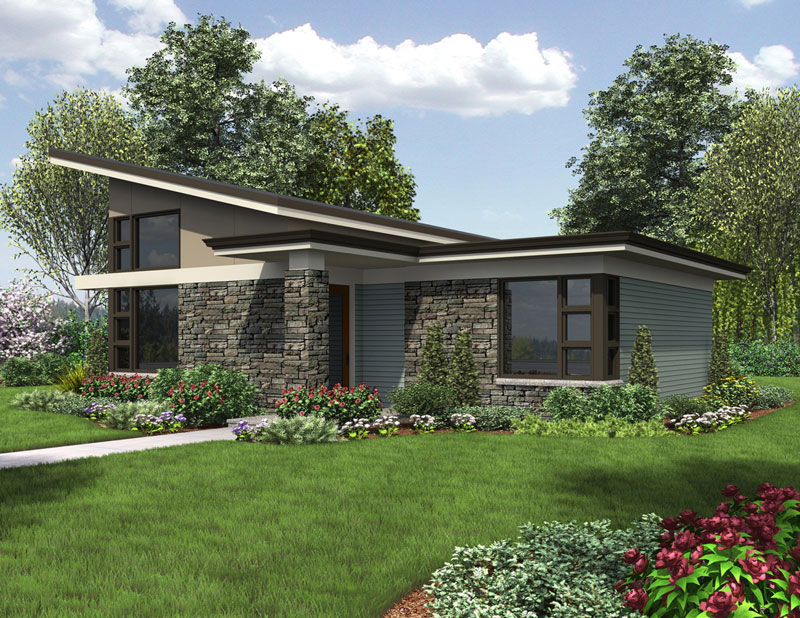This image portrays a 3D generated model of a modern, postmodern house likely designed in the late 2000s to early 2010s. The house features a distinct slanted roof and a facade that integrates stone and brick elements, as well as wooden slats. The entrance, marked by a stone pillar, includes a glass door situated on the left-hand side as you approach via a white walkway. Large, floor-to-ceiling windows dominate the front, offering an open, airy feel. The two-story house is surrounded by a meticulously maintained lawn, vibrant flowerbeds, and lush shrubbery, with cranberry or deep red roses adding a splash of color. The sky overhead is a bright blue, dotted with large, white clouds, enhancing the picturesque setting. This beautifully designed home, with its incredible architecture and inviting landscape, exudes an atmosphere of modern elegance and tranquility.